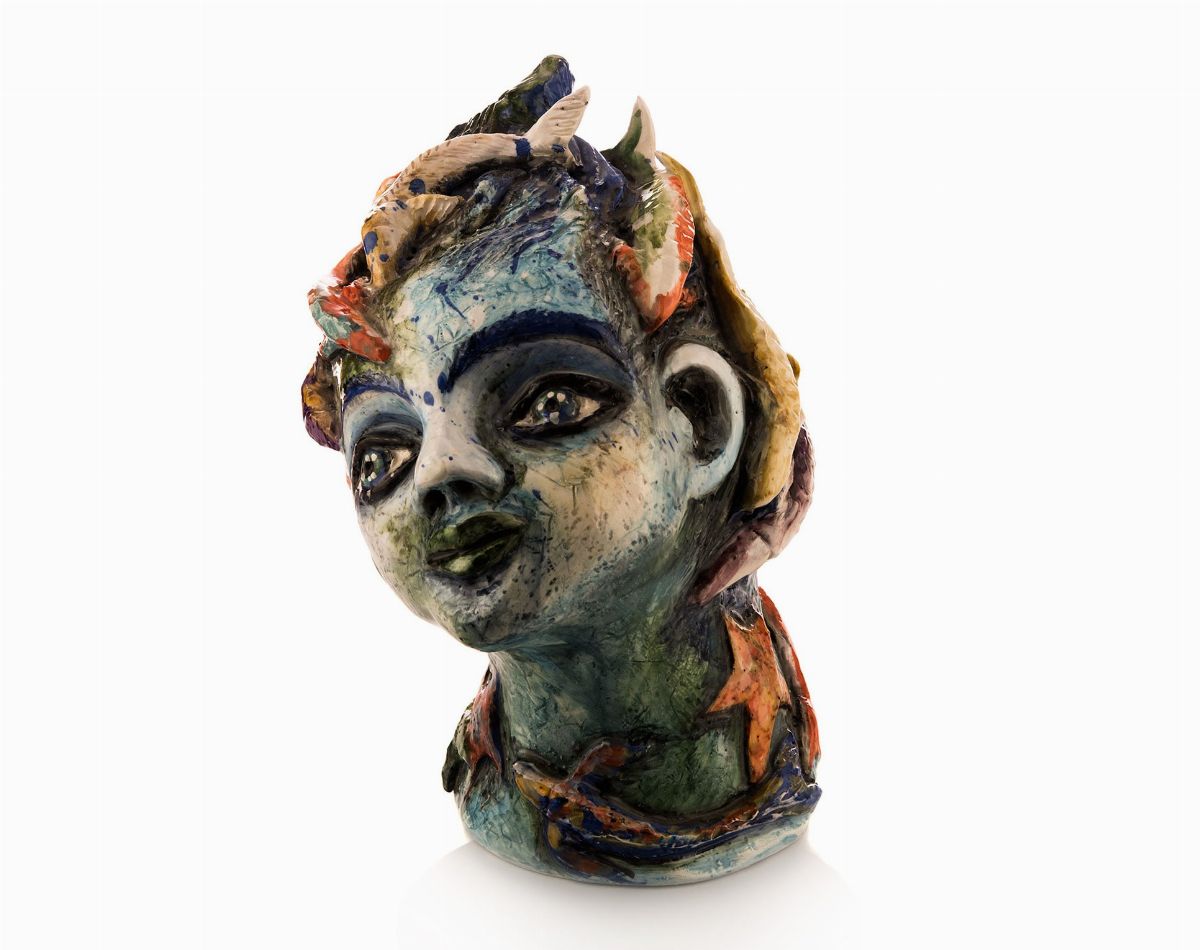This image depicts a professionally crafted, avant-garde sculpture of a woman's head and neck set against a completely white background. The skin features a striking palette of black, green, gray, white, and purple hues, lending an otherworldly and slightly unreal quality to her appearance. Her face is adorned with thick black eyebrows, grayish-blue eyes, and dark lips. She has a pug nose and wears an elaborate headdress that appears to be composed of leaf-like structures and various colorful fish, including an orange starfish that is prominently visible on the right side of her neck. A band or laurel with brown leaves encircles her neck like a necklace. The overall design of the piece evokes a fantastical, almost Medusa-like aesthetic, replacing snakes with vibrant, multicolored fish. She gazes dreamily to her right, which corresponds to the left side of the viewer's perspective. The sculpture combines elements of classical busts with imaginative, avant-garde artistry, effectively merging traditional and contemporary styles.